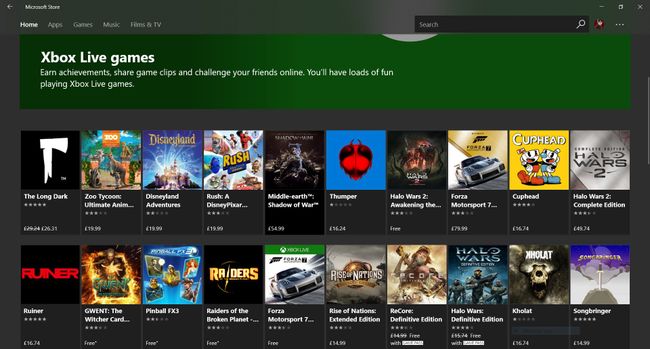The image depicts a bustling interface of the Microsoft Store, specifically tailored for Xbox gaming enthusiasts. Prominently displayed in the top left corner, the title "Microsoft Store" with a left-facing arrow signifies that this is an online webpage. Just beneath this title lies a navigation menu with several options. The 'Home' selection stands out in large white text, flanked by other categories in light gray text including 'Apps,' 'Games,' 'Music,' and 'Films and TV,' directing users to various sections of the store.

In the upper right corner of the page, a sophisticated black search bar featuring light gray placeholder text invites users to find specific content. Adjacent to it is the user profile image, rendered as a red circle, accompanied by an icon of three horizontal white dots which likely opens additional settings or options.

Centrally, a prominent green box captures attention, highlighting Xbox Live Games. It features white text proclaiming, "Xbox Live Games: Earn achievements, share game clips, and challenge your friends online. You'll have loads of fun playing Xbox Live Games." The box also hints at the Xbox logo with a partially visible silhouette in its top-right corner.

Below this callout are two horizontal rows of vibrant video game titles available for purchase. Approximately ten games per row showcase an assortment of genres with titles such as "Disneyland Adventures," "Cuphead," and "Forza Motorsport 7." Each game’s listing includes a vividly colorful box art image, the game's name, a rating out of five stars, and the price, creating an inviting and detailed snapshot of the gaming options available on the platform.